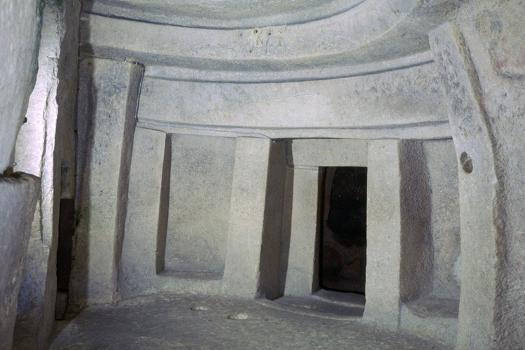This photograph depicts the interior of a cave-like structure carved out of white stone or marble, resembling a grand, ancient architectural space. The image captures both the left and right walls, as well as the ceiling and floor, all constructed from the same white material, possibly white marble, giving the space a monochromatic and seamless appearance. The walls display several rectangular indentations and carvings, suggesting previous architectural elements such as doorways. On the left side, an almost door-shaped rectangle is noticeable but sealed by stone. Further left, at such an angle that a black hole is partly visible, presumably marking an entrance. The middle-right section features a precisely carved rectangular doorway leading into darkness, its sharp, clean lines indicating a meticulous construction process. The overall ambiance hints at an ancient, possibly Roman-era structure, with elements that suggest it may have once been part of a grander, more ornate building, perhaps even resembling an old theater with its rounded, dome-like walls and symmetrical carvings.